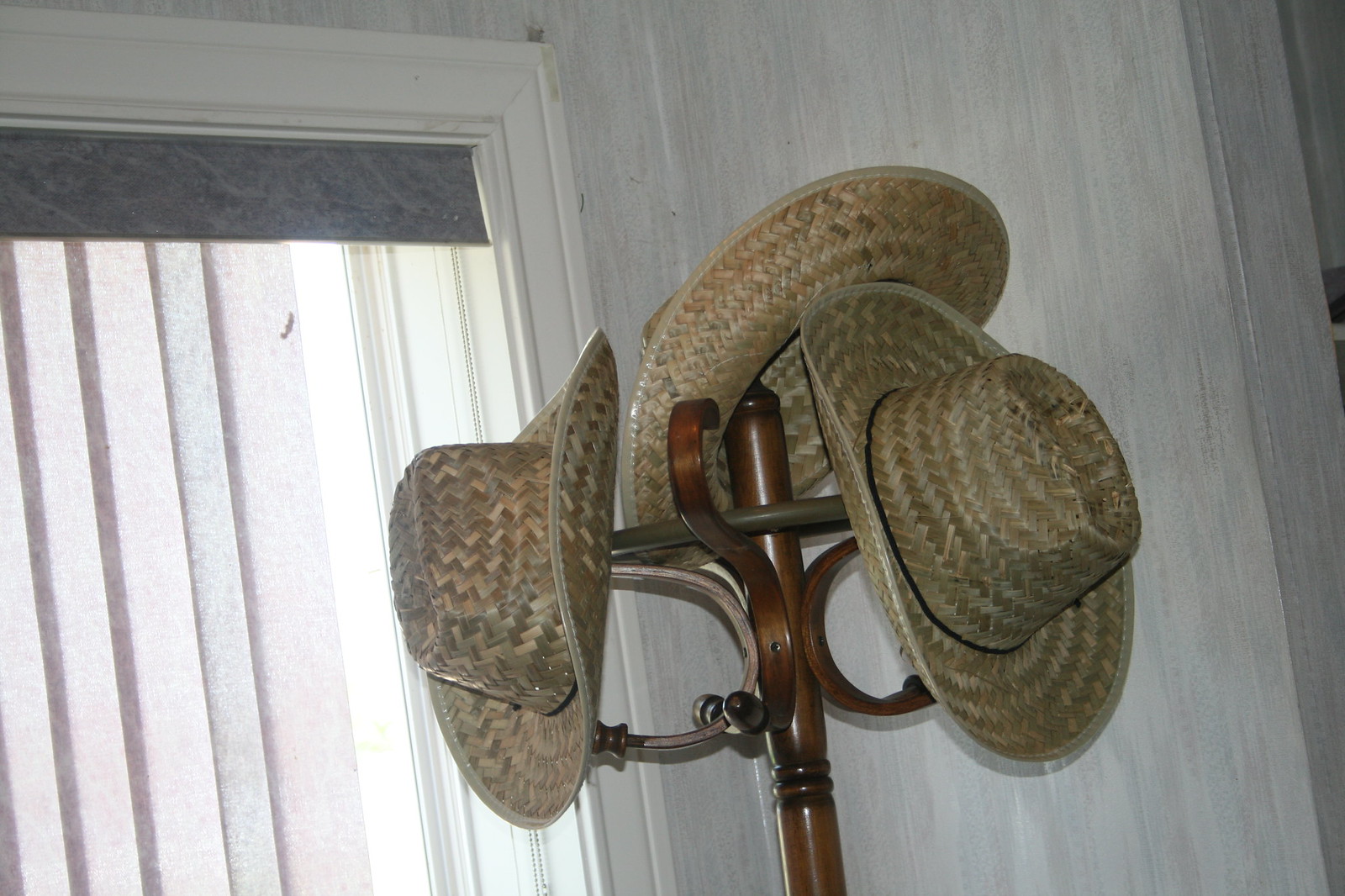This indoor photo captures the corner of a front door entryway adorned with subtle white wallpaper featuring faint gray streaky patterns. The scene is bordered by white trim and a door frame on the left side, and white vertical blinds cover a window or sliding door, letting in a faint stream of light. The focal point is an intricately designed freestanding wooden hat rack with a lathe-turned appearance, complete with a circular ring and four S-shaped hooks. Atop this rack, three straw hats are neatly arranged. These light blondish-tan woven hats, with their flat squash designs, slightly upturned brims, and top indentations, evoke a rustic charm reminiscent of fairground headgear rather than true cowboy hats. One hat perches centrally at the top, its brim curving up to reveal its underside, while the other two balance on either side, showcasing the functional yet decorative prowess of this classic hat rack.